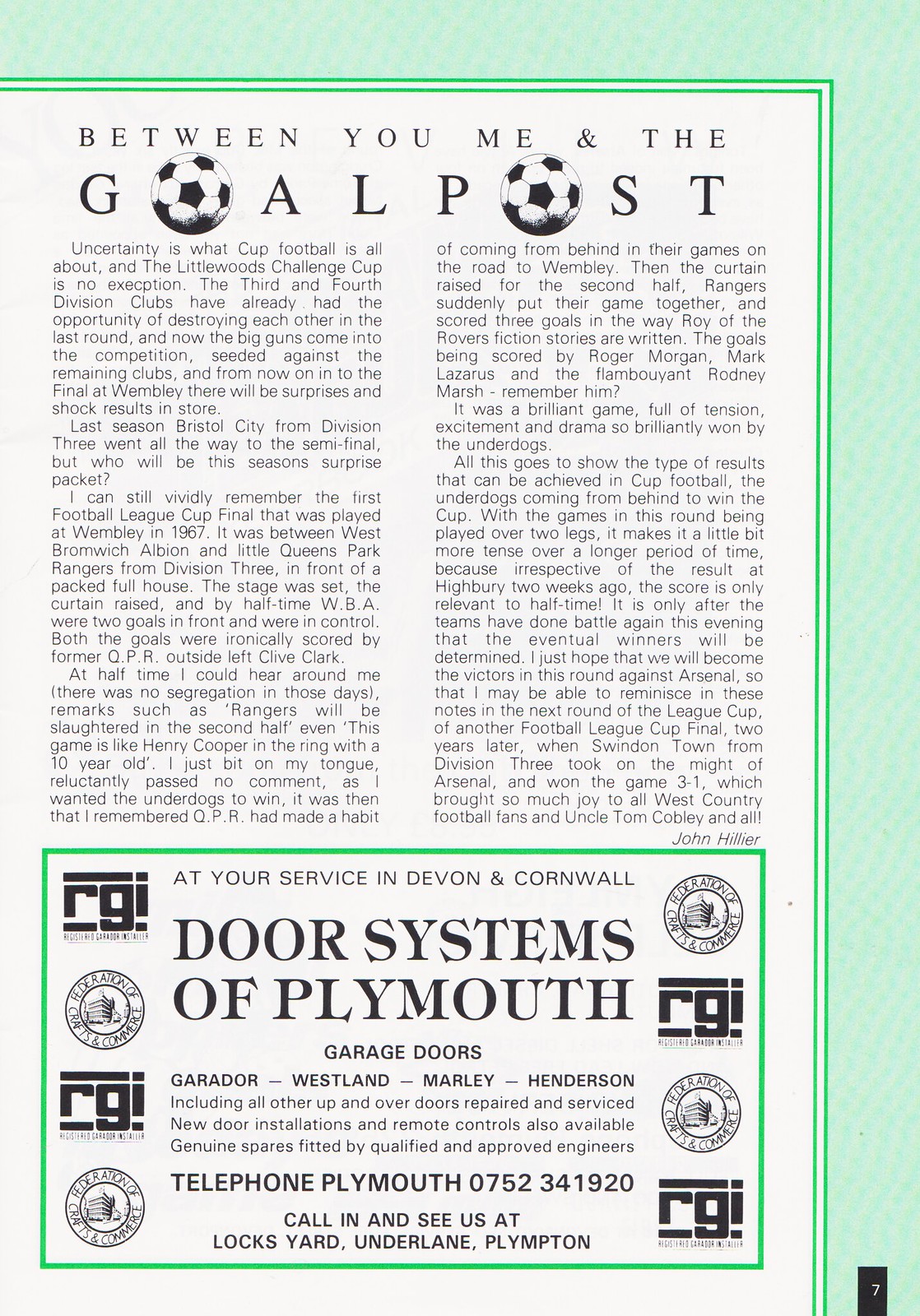The image is a magazine page featuring an article and an advertisement. The page is bordered on the top and right with a checkered green pattern. At the center, the main portion of the page has a white background. The title of the article, written in black font at the top, reads "Between You, Me, and the Goalpost," with the O's in "goalpost" stylized as soccer balls.

The article, consisting of two columns of text, begins with: "Uncertainty is what cup football is all about and the Littlewoods Challenge Cup is no exception. The Third and Fourth Division clubs have already had the opportunity of destroying each other in the last round. Now the big guns come into the competition, seeded against the remaining clubs. From now on into the final at Wembley, there will be surprises and shock results in store. Last season, Bristol City from Division Three went all the way to the semifinal. But who will be this season's surprise packet? I vividly remember the first Football League Cup final at Wembley between West Bromwich Albion and Queens Park Rangers from Division Three. The packed house witnessed West Bromwich Albion leading with two goals by halftime, both ironically scored by former QPR player Clive Clark. Yet, QPR made a comeback in the second half, scoring three goals through Roger Morgan, Mark Lazarus, and the flamboyant Rodney Marsh, showcasing the excitement and drama of cup football."

The text continues to describe more anecdotes and thrilling moments from past cup matches, emphasizing the unpredictability and excitement inherent in the tournament.

At the bottom of the page is a green rectangle containing an advertisement with the text, "At Your Service in Devon and Cornwall: Door Systems of Plymouth," followed by information about garage door repairs, new installations, and remote controls available. The advertisement includes two logos on the left and right sides: "RGI" indicating a Registered Garrador Installer, and a circular logo for the Federation of Crafts and Commerce. The advertisement ends with contact details: "Telephone Plymouth 0752341920. Call in and see us at Locks Yard, Under Lane, Plympton.”